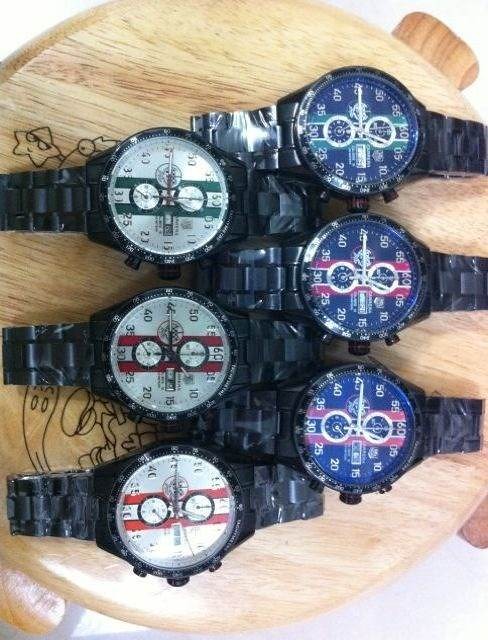This is a detailed photograph taken from a close-up, bird's-eye view, showcasing six wristwatches meticulously arranged on a circular wooden surface, likely a desk. The circular desk has small legs that stick out at the edges. The watches are positioned side by side in a two-by-three layout, where three watches are on one side and three on the other, creating an interlocking design with their faces touching.

Each watch features a black wristband that appears to be made of metal with chain links. The faces of the watches are the focal point, displaying different colors and patterns. The left three watches have white faces, each adorned with vertical stripes: the top one has green stripes, the middle one has red stripes, and the bottom one features orange stripes. The three on the right side have black faces with their own colored vertical stripes: the top one has teal, the middle has red, and the bottom has pink stripes. 

Additionally, there is small black text and clip-art-like figures on the left-hand side of the wooden surface, adding a touch of whimsy to the image. This detailed arrangement highlights both the uniformity and the unique color variations of the watch faces.